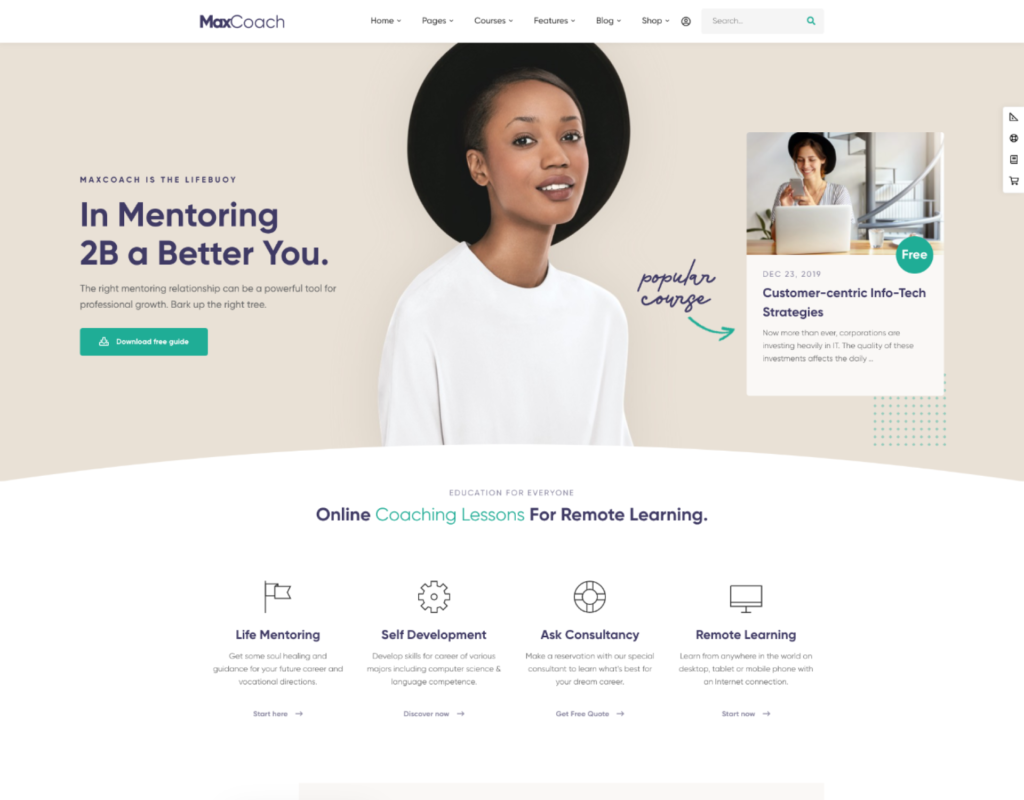**Description:**

The image is a screenshot of the homepage for a website called "MaxCoach." The brand "MaxCoach" is presented as a single word with a stylized "Max" and a classic "Coach." The website has a white navigation bar at the top, featuring menu options like "Home," "Courses," "Features," "Blog," and "Shop," each with a drop-down menu. Towards the right, there are icons for user profile and search, the latter with a green magnifying glass icon.

The main section of the webpage features a beige background. Central to this section is a striking image of a Black woman wearing a wide-brimmed black hat and a white shirt, gazing directly at the viewer. To the left of her, a prominent text reads: "MaxCoach is the lifebuoy in mentoring to be a better you. The right mentoring relationship can be a powerful tool for professional growth. Bark up the right tree." Below this, there's a green button labeled "Download Free Guide."

On the right side is a section titled "Popular Course," which features another Black woman, similarly dressed in a wide-brimmed black hat, seated at a desk and looking at a laptop. The accompanying text reads: "December 23, 2019: Customer-Centric Infotech Strategies. Now more than ever, corporations are heavily investing in IT. The quality of these investments affects the day..."

The overall resolution of the site is poor, which makes some of the smaller text difficult to read.